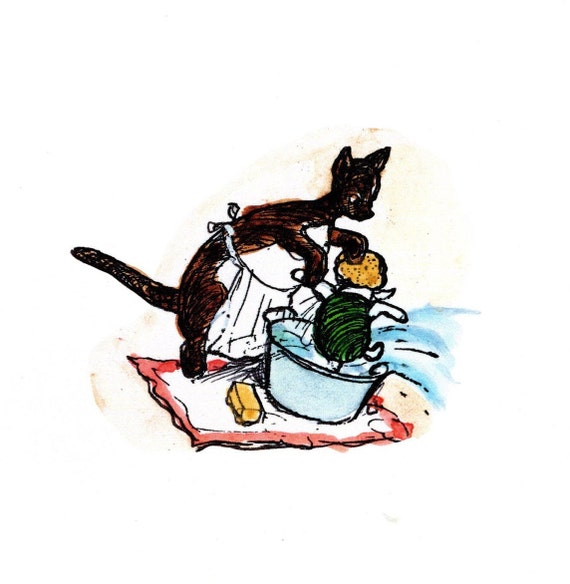The image is a basic, childlike drawing with a square shape set against a translucent background, depicting a cartoonish scene. At the center is a roughly drawn cat, though some interpretations suggest it might be a kangaroo mother, wearing a white apron that starts at her midsection. This character is bent over a large pot full of water, vigorously scrubbing another smaller animal's head using a sponge or loofah. While some believe the smaller animal resembles a pig, others see a kangaroo baby in a green shirt, possibly suggesting a resemblance to Kanga and Roo from "Winnie the Pooh."

The water splashes out of the pot due to the smaller animal’s fussing, creating a messy scene. Nearby, a bar of soap sits on the floor. Both characters are positioned atop a red-trimmed blanket with a white center, against what appears to be a sandy or neutral background. The cat (or kangaroo) has indistinct facial features, contributing to the drawing's crude and unusual appearance.